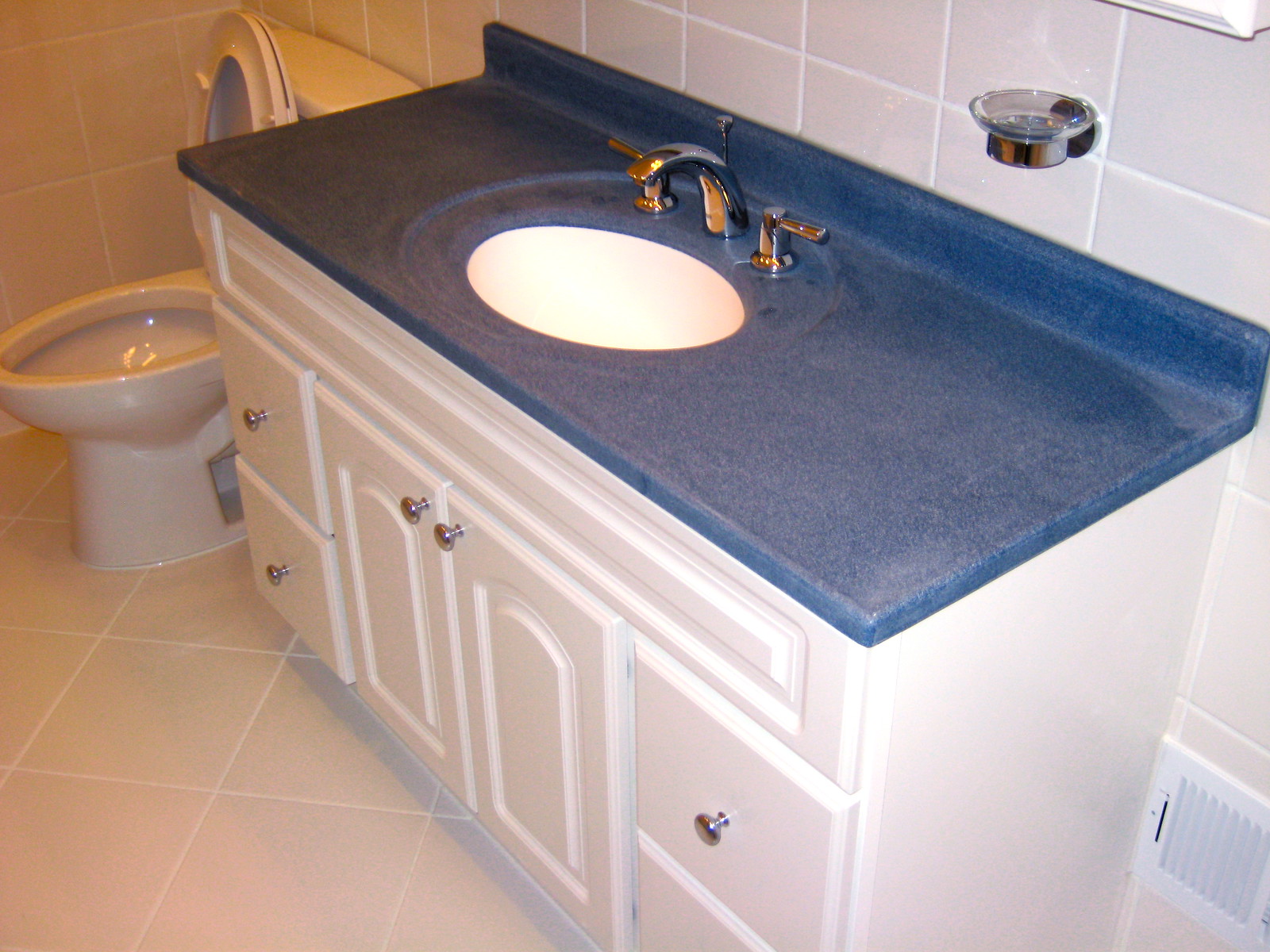The image depicts a pristine bathroom showcasing a clean and modern aesthetic. At its center stands a gleaming white porcelain toilet, with the seat lifted to reveal an empty, shiny interior and a matching white tank. To the right, a sizable black, marbleized countertop featuring a minimalistic design with subtle dots embedded in the material serves as the base for a silver faucet with matching handles. The circular sink is crisp white, providing a stark contrast to the dark countertop. Below, the vanity consists of white wooden cabinetry, viewed from a left-front perspective, with two drawers on the left adorned with silver knobs; twin cabinets in the middle, each with a silver handle; and additional drawers on the right, though the lower drawer handle is obscured from view. Beige tiles with white grout cover both the floor and walls, fostering a cohesive and elegantly neutral tone. A small, silver soap dish is affixed to the wall, complemented by a white vent positioned on the right.